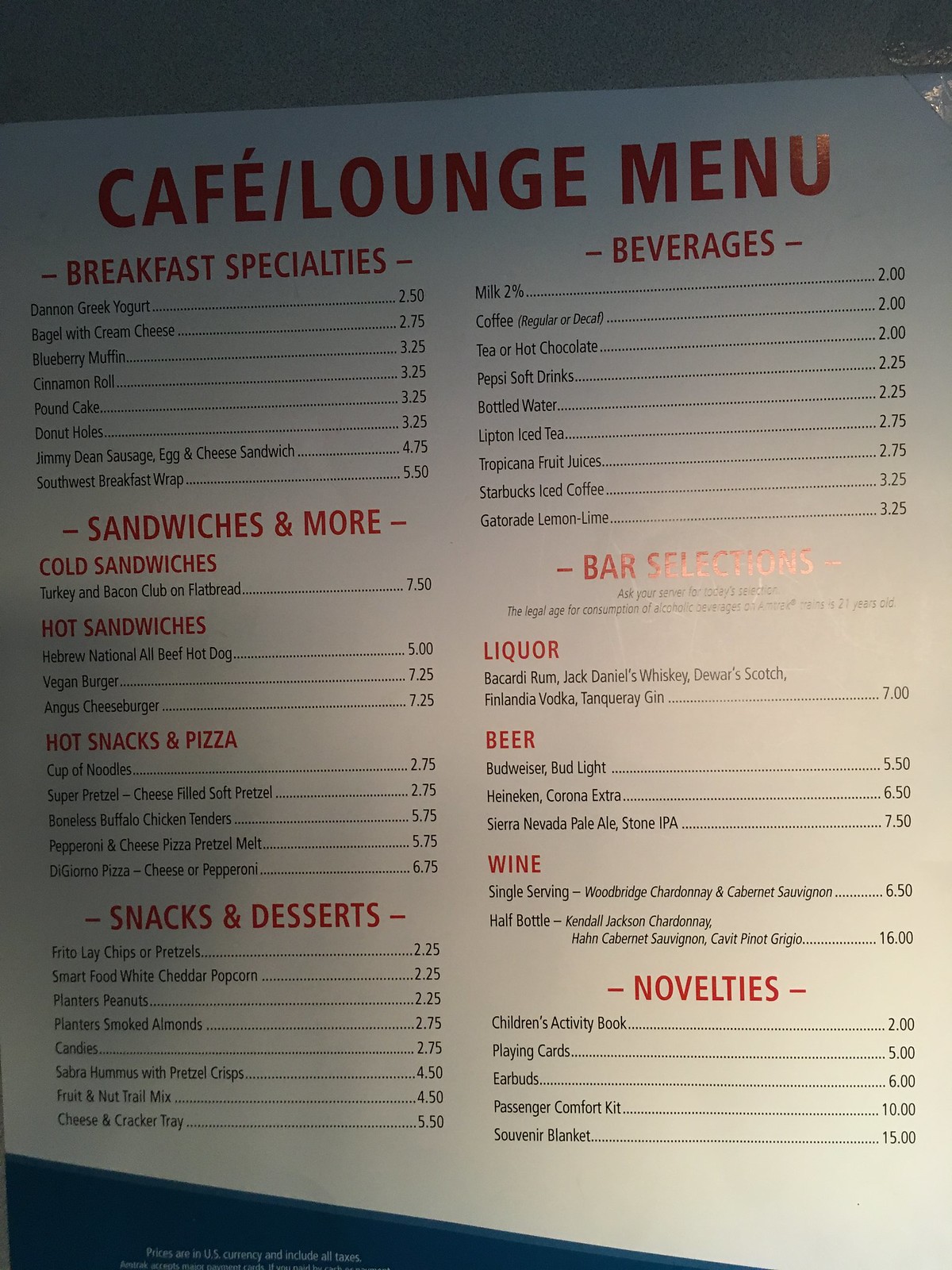**Detailed Descriptive Caption:**

A photo of a white menu with red headings and black text provides a variety of culinary options. The menu's pricing is listed in US currency, although some parts are challenging to decipher. It neatly categorizes its offerings into sections: Breakfast Specialties, Sandwiches and More, Snacks and Desserts, Beverages, Bar Selections, and Novelties.

In the Breakfast Specialties section, the menu features items such as Dannon Greek Yogurt, Bagel with Cream Cheese, Blueberry Muffin, Cinnamon Roll, Pound Cake, Donut Holes, Jimmy Dean's Sausage, Egg and Cheese Sandwich, and a Southwest Breakfast Wrap.

The Sandwiches and More section showcases an assortment of meals, including Cold Sandwiches like the Turkey and Bacon Club on Flatbread and Hot Sandwiches such as the Hebrew National All Beef Hot Dog, Vegan Burger, and Angus Cheeseburger. For hot snacks and pizza lovers, options include Cup of Noodles, Super Pretzel, Cheese Filled Soft Pretzel, Boneless Buffalo Chicken Tenders, Pepperoni and Cheese Pizza Pretzel Melt, and DiGiorno Pizza available in Cheese or Pepperoni variants.

The Snacks section suggests a range of low-priced snacks ideal for those on the go, making the menu a versatile choice for various tastes and preferences.